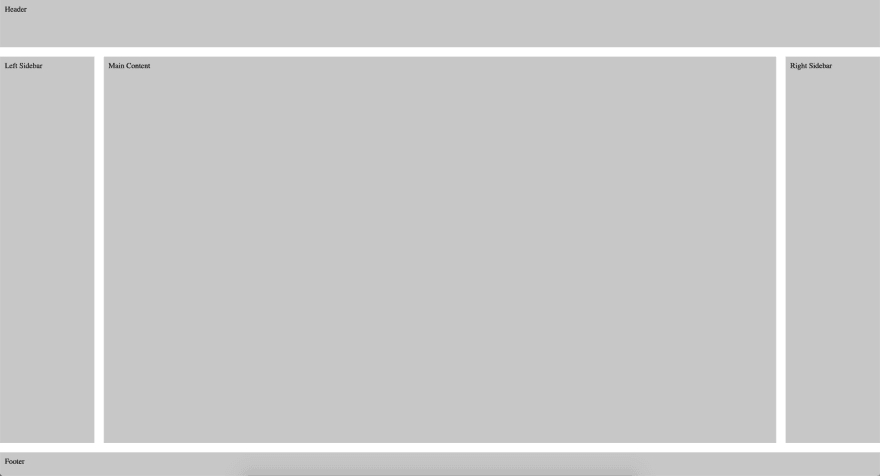This image showcases a landscape-oriented prototype layout for a future website, meticulously designed on a desktop. Featuring a clean white background, the layout elegantly divides the potential website into distinct sections using shades of grey. At the top, a horizontal light grey bar is labeled "Header" in the upper left corner, demarcating the website's beginning. The central area is segmented into three distinct sections: a narrow "Left Sidebar," a more expansive "Main Content" section in the middle, and another narrow "Right Sidebar." Each section is clearly marked with slightly darker grey text for easy identification. Below these sections, a long, slim horizontal area labeled "Footer" completes the layout, also marked in the upper left corner. Overall, the layout comprises five sections, organized into three primary segments, effectively displaying the website's structural blueprint.